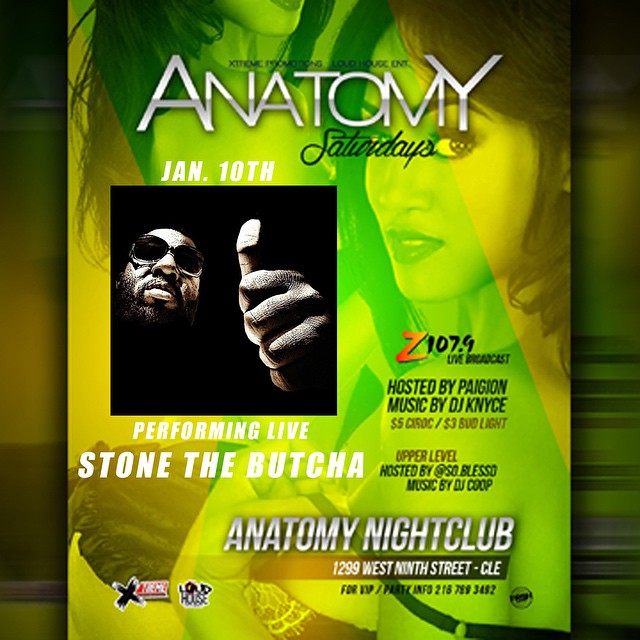This is a portrait rectangular poster advertisement for "Anatomy Saturdays." Centered at the top, the word "ANATOMY" appears in a stylized, all-caps font with the 'A' and 'Y' larger than the rest of the letters. Beneath it, "Saturdays" is written in italicized black text. The bright background features overlaid green and yellow hues, with images of two women. The woman on the right, with brown hair, lipstick, big eyes, and curvy eyebrows, looks directly at the viewer while bearing a seductive expression and pulling her bra off her shoulder. To her left is the bottom half of another woman's face framed by long, curly hair. Both appear attractive. 

Overlaying the background is a black square featuring an African-American man with a mustache, beard, dark glasses, and a thumbs-up gesture. Above him, in white text, it reads "Jan. 10th," and below, "Performing Live, Stone the Butcher," likely identifying the man as the performer. To the center-right is the Z107.9 logo, indicating the sponsor. The text also mentions "Hosted by Pagion, Music by DJ Knice (K-N-Y-C-E)." At the upper level, it denotes hosting by "At So Blessed," with music by "DJ Coop." Beer prices are advertised as "$3 Bud Light" and "$5 Ciroc."

At the bottom, the poster lists "Anatomy Nightclub, 1299 West 9th Street, CLE" as the venue's address, presumably in Cleveland. For VIP and party information, a phone number, "216-789-3492," is provided. Additional logos include one resembling a black "X" with a red banner and another with a scribble-like "Loud House" text.